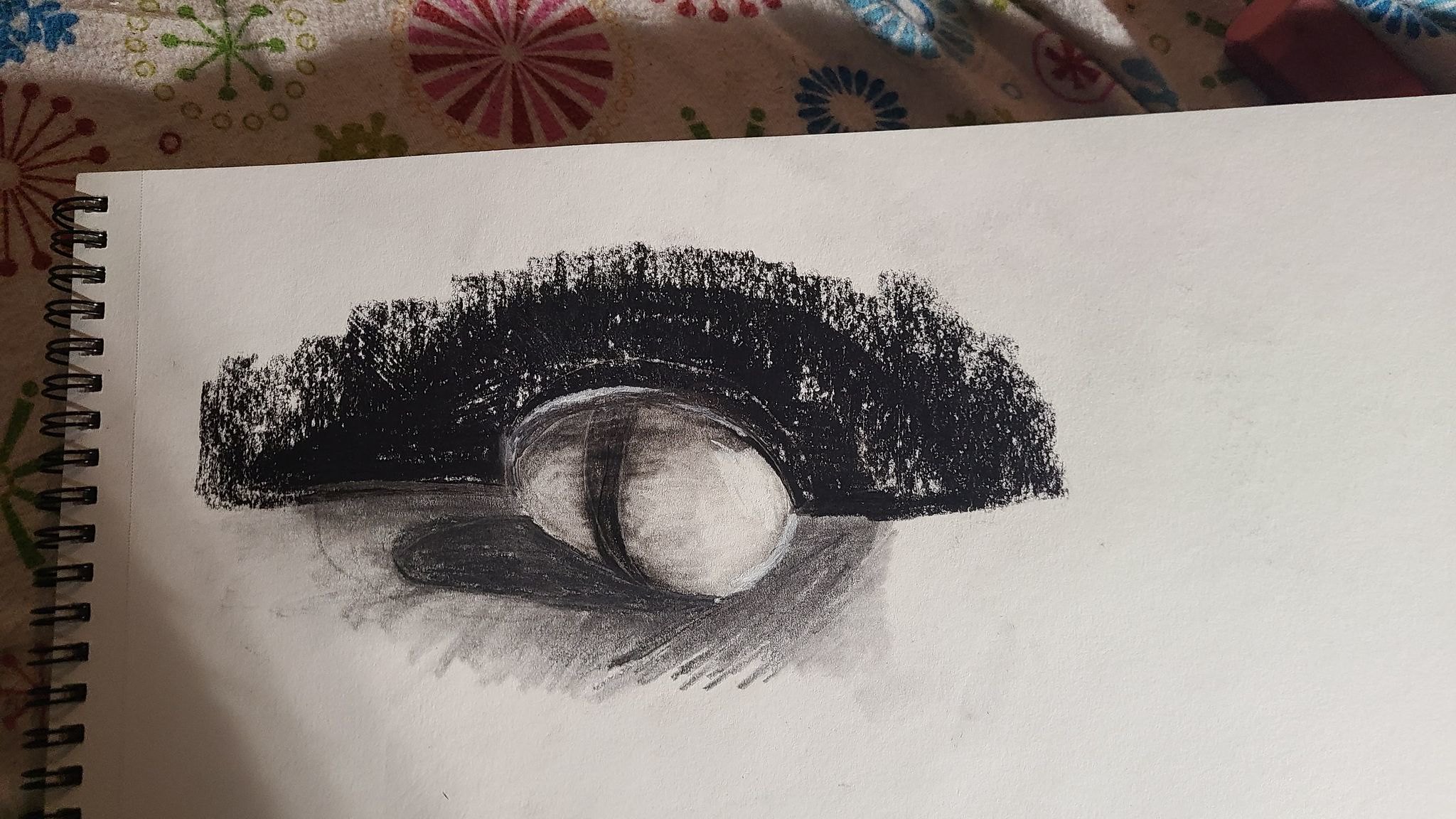In this horizontally elongated rectangular image, we see an open artist's sketch pad with the black binding running vertically along the left edge. The pages are an off-white cream color, creating a warm and inviting canvas for the artwork. On the page, a darkly penciled sketch captures our attention. At the center of the composition, there appears to be an oval or egg-shaped area that is significantly lighter than its surroundings, likely depicting a lake. Encircling the upper half of this lake is a mountain, shaded in dark pencil with subtle touches of white to potentially represent snowfall. Emerging from the peak of the mountain are numerous treetops, sketched impressionistically rather than adhering to strict realism, adding to the abstract quality of the drawing. The overall scene exudes an aura of tranquil wilderness, though it remains open to interpretation. Notably, there is no visible signature from the artist on this piece.